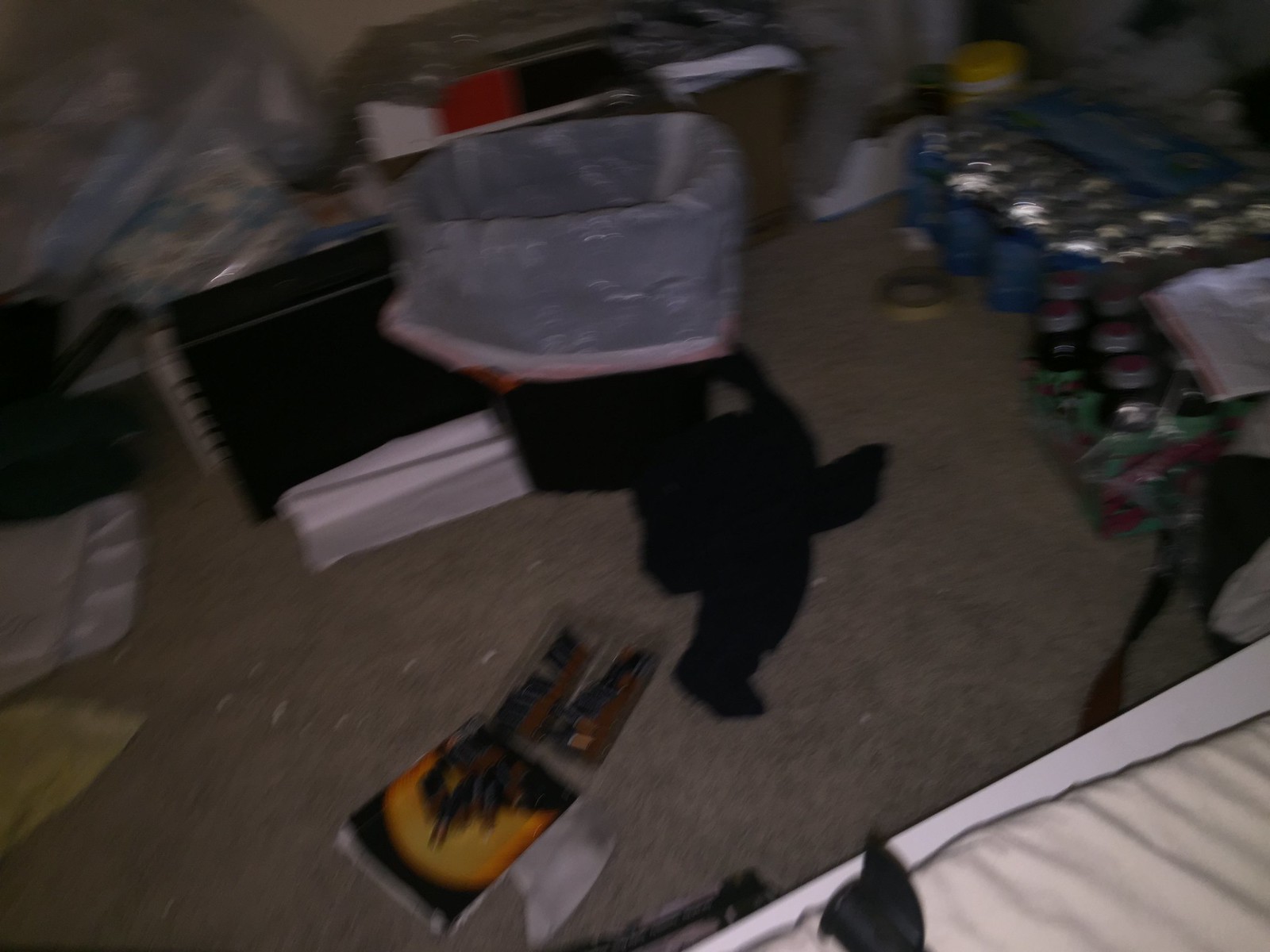The image shows a cluttered room with a grayish, dirty carpet. A small, brown trash can with a white bag is positioned center-left amidst the disarray. On the right side, a torn-open case of Arizona iced tea and a large 40-pack of water bottles lie haphazardly. Nearby are scattered magazines, various papers, and a round container with a yellow lid, likely for sanitizing wipes. Beer cans in blue and red stack up along the right wall, leading down to a busted CD case with black album artwork featuring a bright orange sun. A disheveled white mattress occupies the bottom right corner, partially covered by what seems to be a bed sheet. Dirty black clothes and random plastic containers add to the overall messiness, suggesting a neglected, perhaps dorm-like environment.